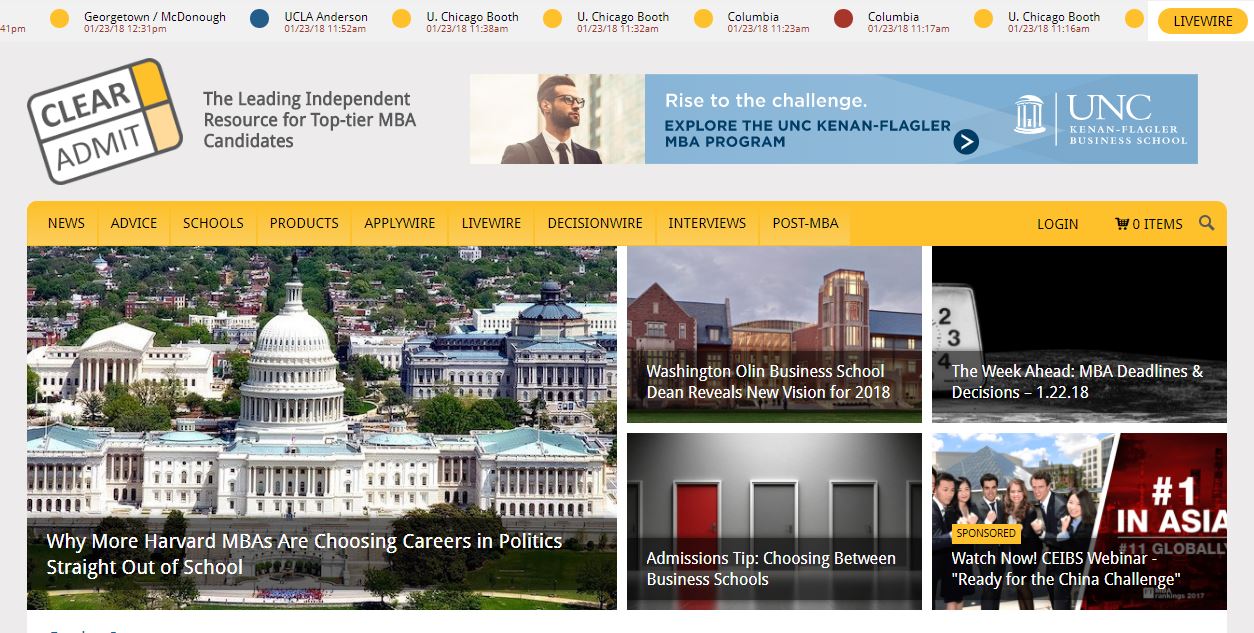This image is a detailed layout of various graphical elements and text. 

Starting from the top left, there is a grey rectangle featuring:
1. A yellow circle containing black text, followed by a line of additional black text and red text below it.
2. A blue circle with black text to its right and red text beneath it.
3. Another five yellow circles, each with black text beside them and red text underneath.
4. A red circle with a black or dark blue word next to it and red text below.
5. A yellow circle followed by black text and red text underneath.
6. A final yellow circle followed by a yellow oval containing a single word.

Further down, there is a tag-like graphic in a mix of orange and light orange, outlined in black with a black horizontal line through its middle, labeled "clear, admit." Words follow this tag.

Adjacent to these circles and tags is:
- A photograph of a man.
- A light and darker blue rectangle containing the text, "Rise to the Challenge, explore the UNC," followed by an unclear word, and "NBA programs."
- A dark blue circle with a white right-pointing arrow and a UNC logo.

Below this section is a long yellow tab with multiple small headers: "news, advice, schools, products, apply," another unclear word, "interviews," and another unclear word.

On the right-hand side:
1. The words "log in" next to a symbol, "zero items," and a magnifying glass icon.

Underneath these elements is:
- An image of the US Capitol building, overlaid with a semi-transparent grey rectangle that reads, "Why more Harvard MBAs are choosing careers in politics straight out of school."
- An image of some buildings with a smaller grey semi-transparent rectangle with undecipherable text.
- An image of a room with multiple grey doors and one red door, overlaid with another semi-transparent grey rectangle containing words.
- An element featuring an icon resembling a clock on the left with a grey semi-transparent rectangle to its right.
- An image showing people on the left and a red section on the right that reads "number one in Asia."
- A yellow rectangle with a word, followed by another grey semi-transparent rectangle containing text. 

This image is structured to present various topics and categories visually, using colored circles, rectangles, and semi-transparent overlays to organize the information.